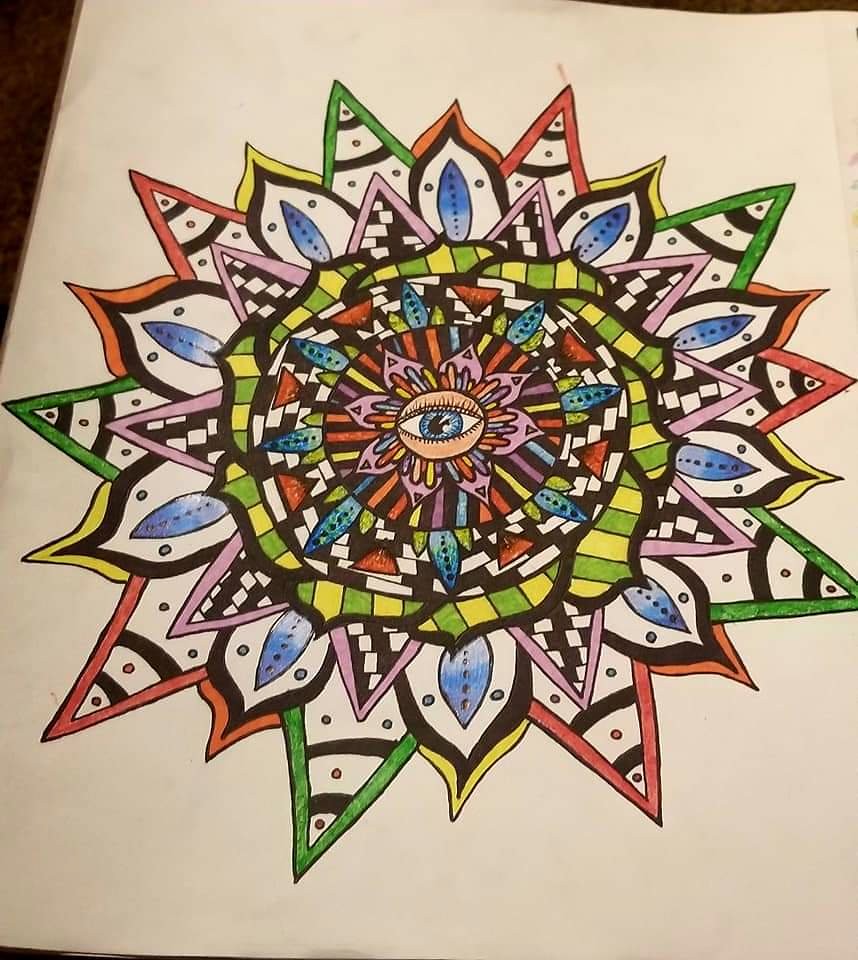This is a highly detailed and colorful drawing on white paper, resembling a psychedelic, flower-like geometric pattern. At the center of the image is a blue human eye with black eyelashes, set within a larger circular shape outlined in brown, giving it a realistic eye-like appearance. Radiating from this central eye are pointy triangles of lilac color, interspersed with colored lines ranging from red, green, orange, pink, to yellow and blue. These lines extend back towards the eye and outward, creating a dynamic flow.

Surrounding the eye, bright and intricate geometric patterns emerge in shades of red, yellow, purple, and blue, some arranged in a mosaic pattern. Midway through the design, there's a layer with green and yellow parts that add to the vibrant complexity. Some sections feature black and white checkered patterns, along with black wavy designs around certain petals.

Further out, a circle of geometrical shapes in red, blue, white, and brown is followed by a circle with curvy edges in yellow and green. The outermost edges of the design display pointed tips reminiscent of poinsettia leaves in varying colors of green and red, all set against the white paper background with brown lines running across them. The detailed patterns and the rich variety of colors suggest a blend of symbolic and random artistic elements, making the entire image appear as a stunningly elaborate, flower-like, psychedelic artwork.